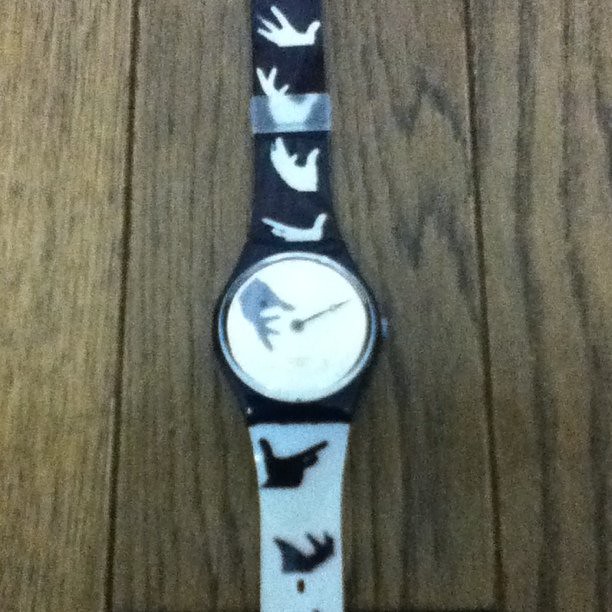This slightly blurry, square-shaped image features a rustic wooden hardwood floor as its background. Centrally positioned, a watch lies vertically across the frame, with both its ends cut off, revealing only a portion of the watch's band. The band in the foreground is white, showcasing two distinct hands with fingers spread in different positions. In the background, further from the viewer, the band is black and depicts four hands arranged in varied positions. A clear strap, intended for threading the other side through, is visible. The watch face itself is white, displaying one hand reaching down from the top and another black hand indicating time. Unfortunately, the numerals on the watch face are obscured due to the blurriness of the image.